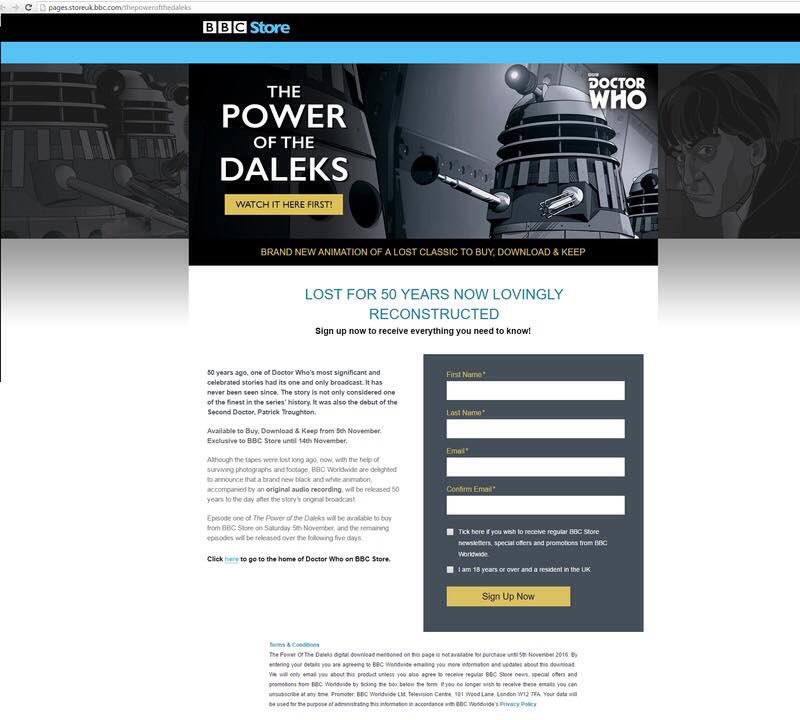The desktop screenshot captures the BBC Store website, prominently displaying "BBC Store" in blue text alongside the BBC logo in a banner at the top. The focal point of the webpage is an advertisement for the iconic sci-fi show Doctor Who, specifically featuring the robotic alien species known as the Daleks. On the right side of the page is a black-and-white illustration of a Dalek, which resembles a scrap-metal version of R2-D2. The left side of the advertisement reads, "The Power of the Daleks" in bold white text, followed by "Watch it here first."

The advertisement continues with the text: "Brand new animation of a lost classic to buy, download and keep. Lost for 50 years, now lovingly reconstructed. Sign up now to receive everything you need to know." Below this, there is additional, smaller text that is unreadable.

On the right side of the webpage, there is a sign-up form prompting users to enter their name, email address, and confirm their email. It also includes checkboxes for additional options and a sign-up button, inviting visitors to subscribe for more information and access to the newly animated Doctor Who content featuring the Daleks.